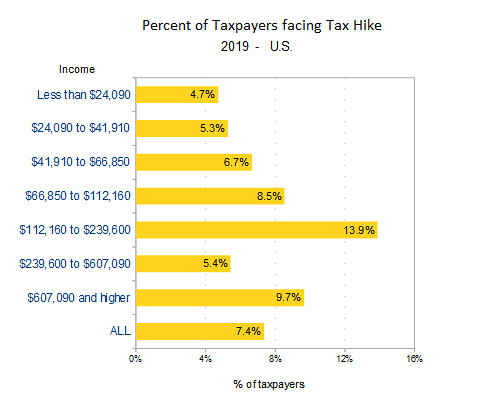The image displays a horizontal bar chart titled "Percent of Taxpayers Facing a Tax Hike 2019, U.S." on a white background with headings in black. The chart illustrates the percentage of taxpayers within various income brackets who are projected to face a tax increase. The bars, colored in yellow, represent these percentages, while the income brackets are listed on the left in blue font. 

Starting with incomes less than $24,090, 4.7% of taxpayers in this bracket face a tax hike. For those earning between $24,090 and $41,910, 5.3% are affected. Taxpayers with incomes from $41,910 to $66,850 see a 6.7% increase. The range from $66,850 to $112,160 faces an 8.5% hike. The most notable group, those making from $112,160 to $239,600, face the highest percentage increase at 13.9%. Interestingly, higher income brackets see lower percentages; for $239,600 to $607,090, 5.4% of taxpayers face a hike, and for incomes above $607,090, 9.7% are affected. Lastly, an overall average for all taxpayers shows a 7.4% rate. The values at the bottom range from 0% to 16%, corresponding to the scale of tax increases.